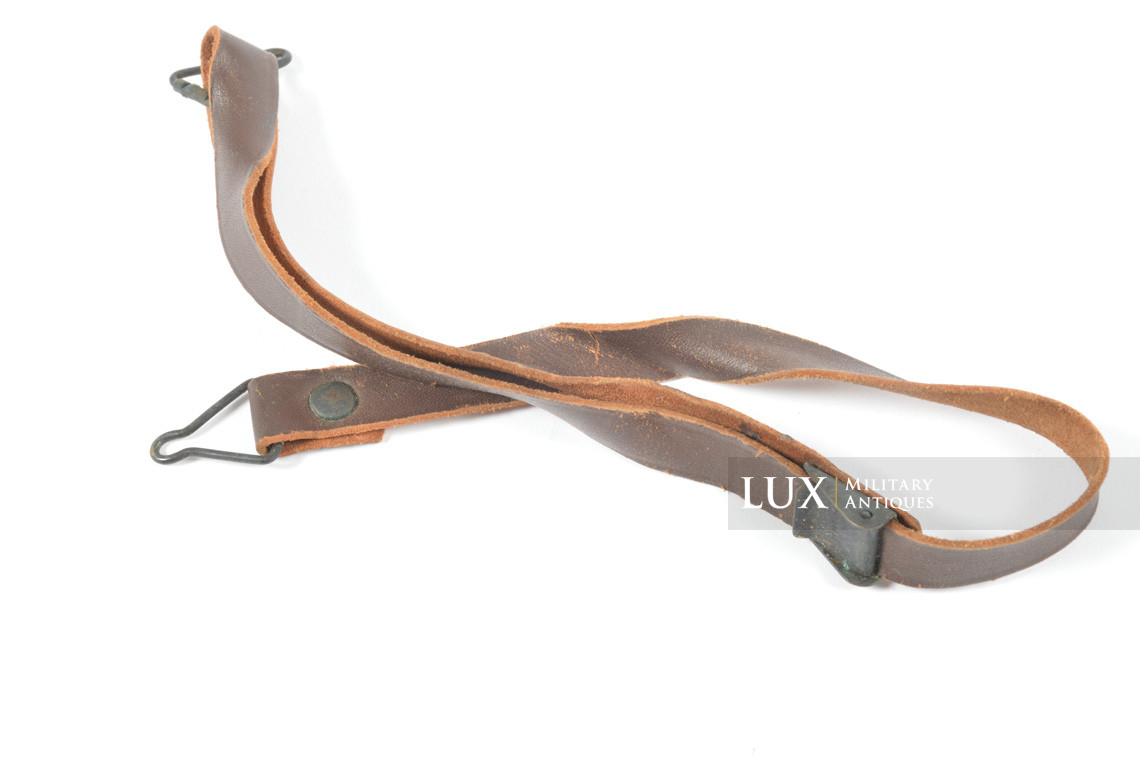The photograph features a single worn leather strap set against a white background. The dark to medium brown leather has untreated edges and shows signs of wear, including a noticeable kink where it has been folded too long. This strap is fitted with metal loops at both ends, resembling cowbell-shaped clips, suggesting it could be part of a suspender or a military accessory. The interior side of the strap has a rough, lighter brown leather texture. Midway along the strap, there is an adjustable buckle mechanism, which can be easily flipped up to modify the length and then locked into place. The image also includes a transparent gray text box situated at the bottom right, containing the text "LUX" in white capital letters, followed by "military antique," indicating the item may be of military origin.